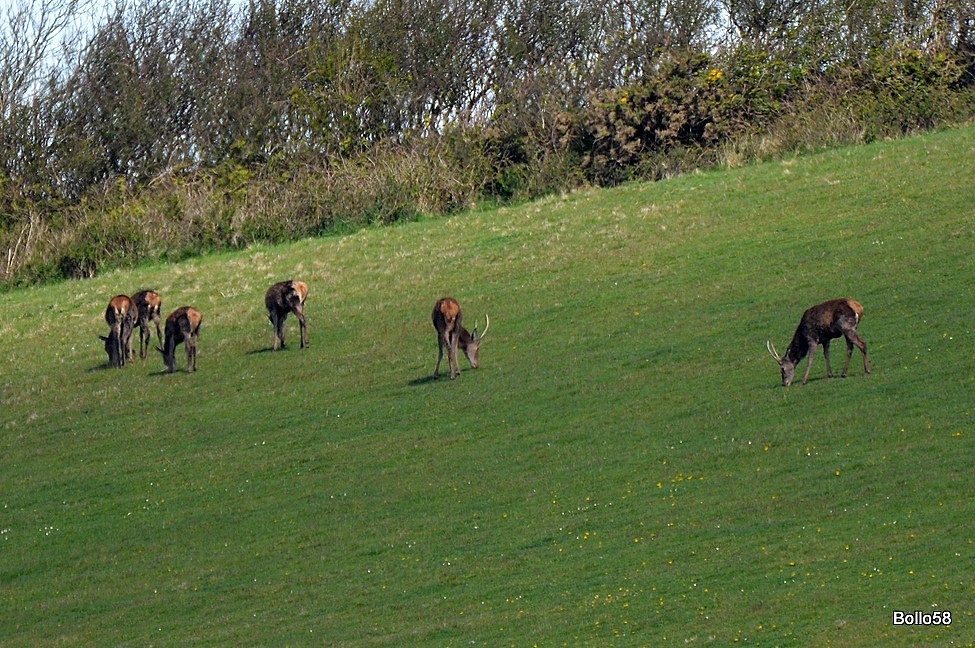In this outdoor photograph, a small herd of six antelope-like animals grazes on a slightly inclined grassy meadow under a bright sun. The lush green grass is dotted with occasional white and yellow flowers, suggesting a vibrant natural setting. The animals are scattered across the photograph; three of them are grouped together towards the left, their heads down as they graze. Another antelope stands to the right of this group, walking towards the center of the image. Near the center, one antelope stands alone, also grazing, while the far-right edge of the photograph features a solitary antelope with its head down, viewed in profile. These animals are brown with black-spotted faces and small horns, resembling deer or antelope. In the background, a line of small, thin trees and shrubs follows the contour of the incline, their dark faded leaves slightly swaying, hinting at a gentle breeze. Above this, the sky is a light blue. In the lower right corner of the image, the text "BALLA58" or "BOLLO 58" is visible.